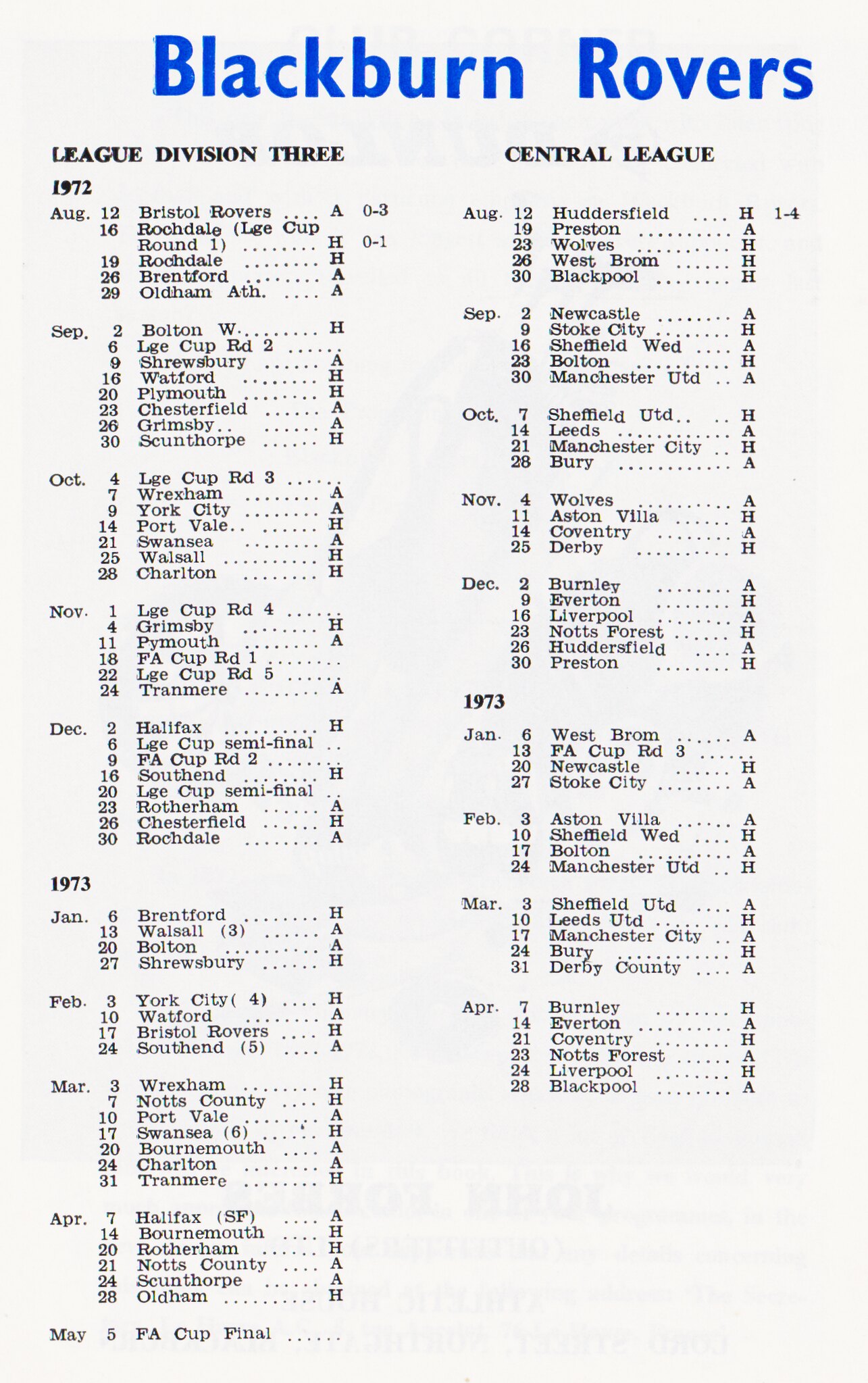This photograph captures a page from a sports program for the Blackburn Rovers, set against a white background. The top of the page features the title "Blackburn Rovers" in large blue letters. The page is divided into two vertical columns: the left column is titled "League Division III" and the right column "Central League." Each column provides a detailed schedule for the years 1972 and 1973, broken down by month from August through May. Within each month, the page lists specific game dates, the opponent clubs, and indicates whether each game is a home ('H') or away ('A') fixture. This organized layout offers supporters an at-a-glance view of the team's upcoming games.